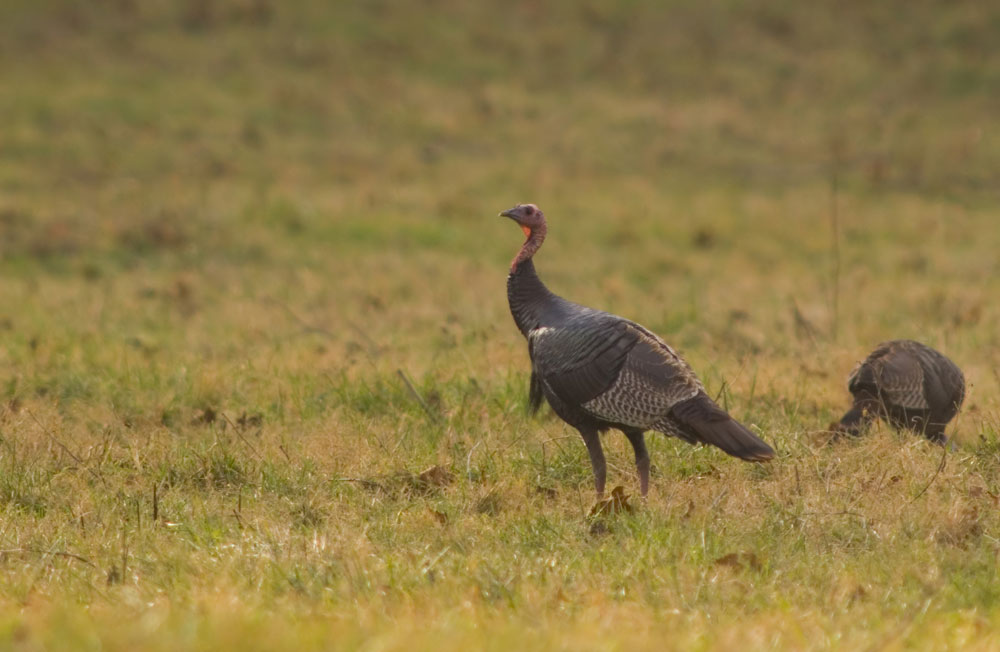The image captures a nature scene featuring two vultures in a grassy field scattered with sticks and leaves. The primary vulture, positioned slightly right of center, has a purplish head and a predominantly black body with some grayish feathers. This bird appears to be gazing toward the left. Just to the right, another vulture is visible, its back turned toward the viewer, bending down as if pecking at something on the ground. The field is a mix of green and brown grass, with brighter patches interspersed with tan and darker hues. The foreground and upper background of the image are slightly blurred, creating a slight depth-of-field effect.